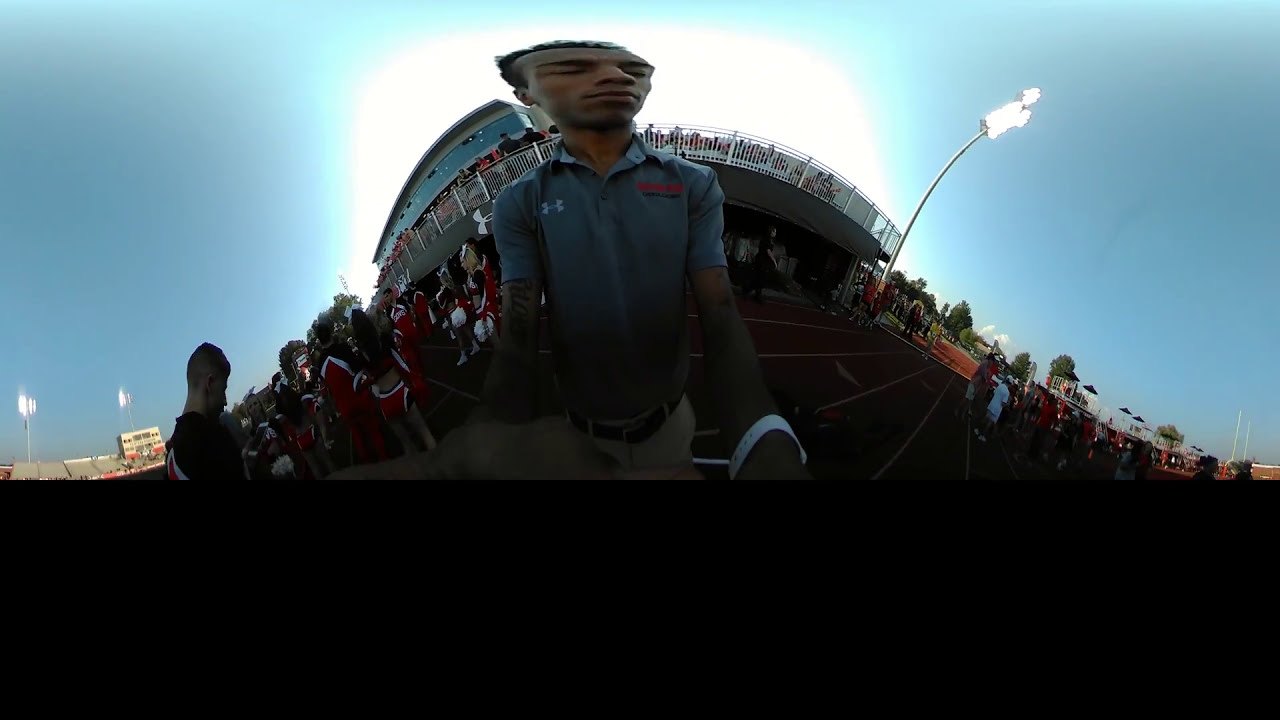The color photograph captures a distorted, almost panoramic selfie of a dark-skinned man at what appears to be a track and field or football event. The man, prominently positioned in the center, appears elongated due to the image’s warp. He is wearing a gray, collared polo shirt with indistinct red and white lettering, possibly with an Under Armour logo. Visible on his left wrist is a white band. Surrounding him, over his right shoulder, is a group of cheerleaders dressed in red and black uniforms, along with one male cheerleader in a black shirt. Over his left shoulder and further behind, there are more people and some people seated in both occupied and empty stands. In the background to the right, there stands a large light fixture, framed against a clear blue sky and verdant trees. The brown track underlines the scene, and the presence of a nearby building with a white railing suggests a stadium setting. The overall atmosphere hints at a lively sporting event in progress.